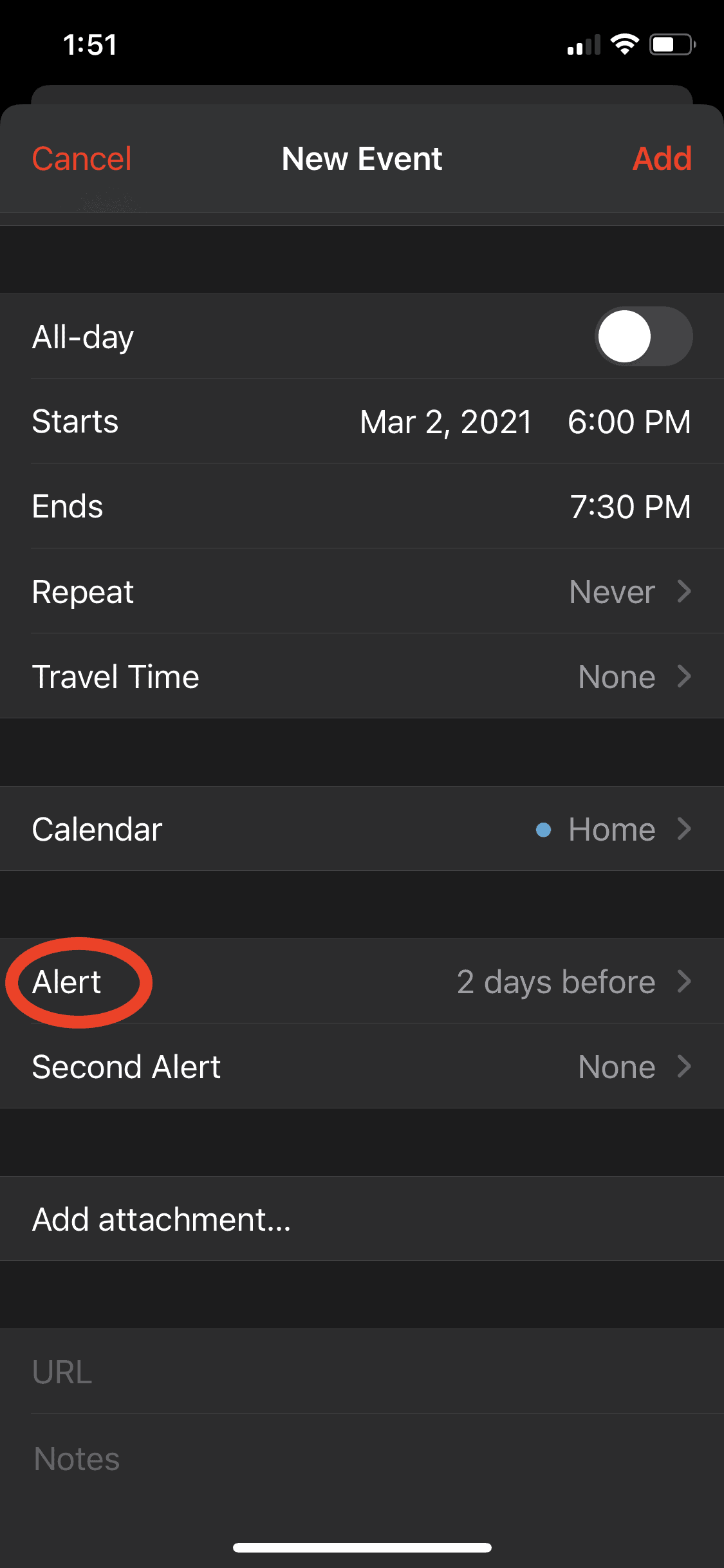This image is a screenshot of a smartphone displaying a "New Event" screen in dark mode. The background is black, providing a contrast to the white text. 

At the upper left corner, the current time is shown in white as 1:51. On the upper right-hand corner, the icons for the battery (approximately half-charged), Wi-Fi, and wireless signal are visible.

Beneath these icons, a slightly lighter, very dark gray banner stretches across the screen. The center of this banner features the text "New Event" in white, while the words "Cancel" and "Add" are displayed in red on the left and right sides respectively.

The screen then displays a section with multiple options, set against a very dark gray background. The text in this section is all in white. On the left, there is a column with options labeled: "All Day," "Starts," "Ends," "Repeats," and "Travel Time." 

Corresponding to the "Starts" label on the right side, the date and time "March 2nd, 2021 at 6 p.m." are displayed. Further down, another rectangle labeled "Calendar" is seen, followed by one labeled "Alert." A red oval has been drawn around the word "Alert."

Beneath this, the label "Second Alert" is visible, and near the bottom of the screen, another rectangle contains the text "Add Attachment" in white.